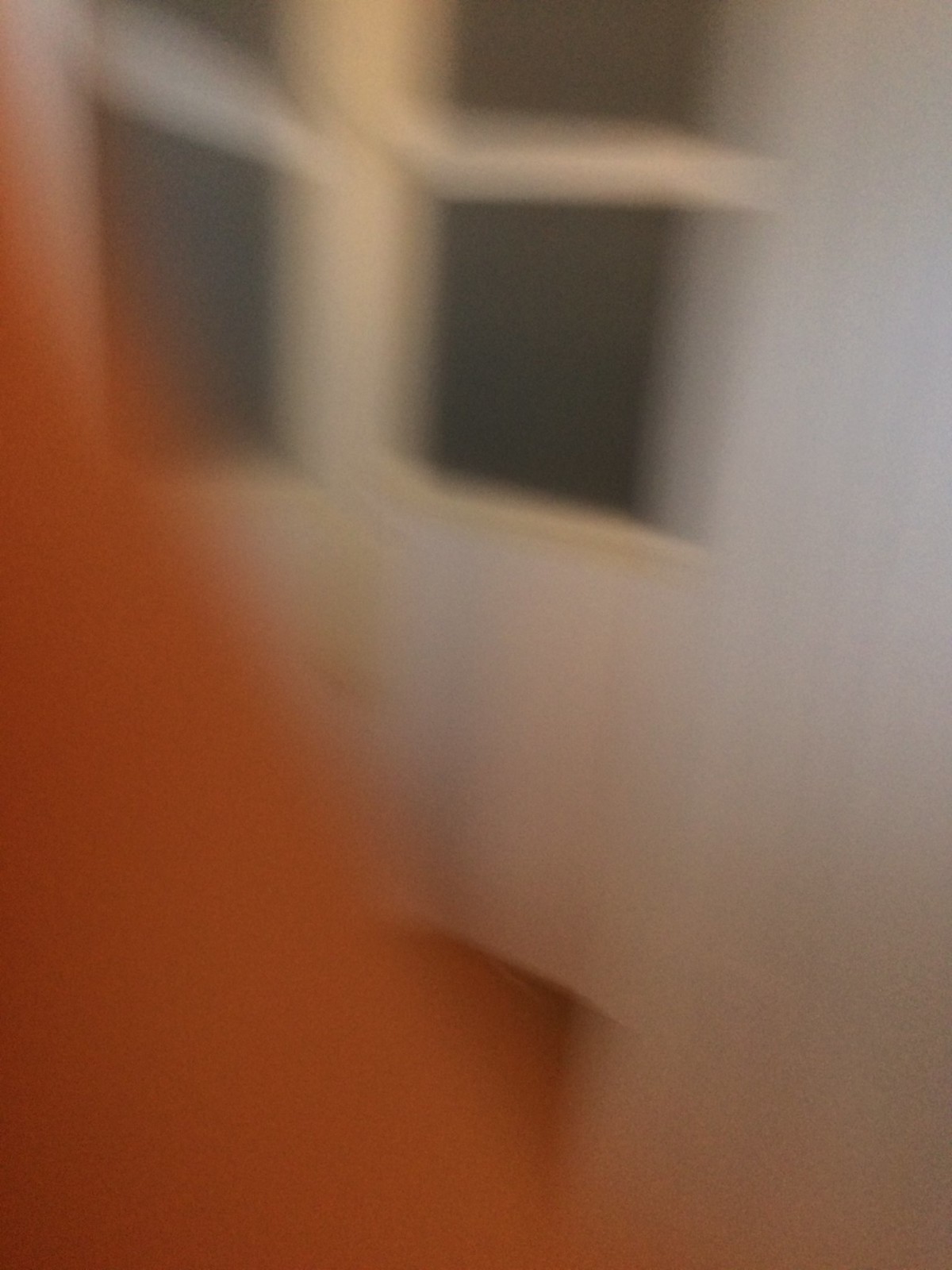The image features a significantly blurred scene dominated by an interplay of whites and deep oranges. In the background, a white setting is partially discernible, interrupted by what appear to be two dark, square shapes. These squares are bisected by white lines, suggesting the presence of a window or similar structure. The left side of the image is saturated with a rich, deep orange hue, creating a stark contrast against the white backdrop. Despite the lack of clarity, the dominant colors of white and orange, punctuated by the two black squares, form a distinct and visually intriguing composition.